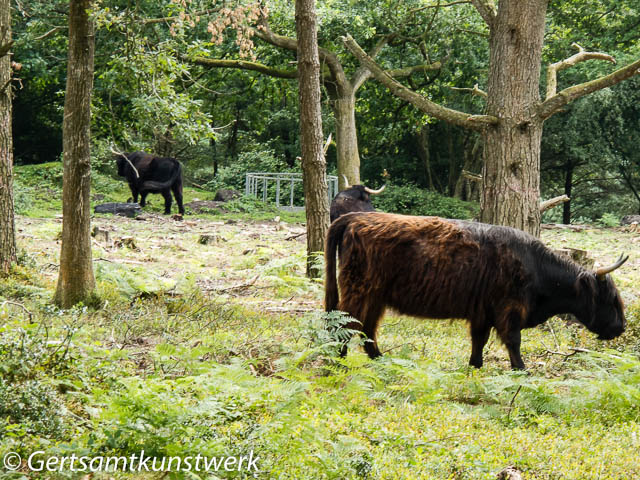In the scene depicted, there is a lush, verdant clearing within a wooded area, possibly part of a nature reserve. The ground is covered in an abundance of green grass and weeds, enhanced by the dense foliage of brown-trunked trees that extend up, their leaves melding into the top third of the image. Three brown and light brown bovine creatures, which resemble buffalo or oxen, are seen grazing calmly on the greenery. Positioned within the frame, one animal stands in the back left, another is right in the middle, and the most prominent figure is closer to the right side of the image. This foremost bovine is distinguished by its lighter hindquarters and darker shoulders and head. In the background, partially obscured by the trees, there is a white, round structure that appears cage-like, possibly indicating a water source or another feature typical of a nature reserve. The animals appear undisturbed by their surroundings and human presence. Finally, in the bottom left corner, there is a logo that reads "© Sam Tickoon's werk" or "© Gert Sam Tungstwerk," marking the photographer's copyright.